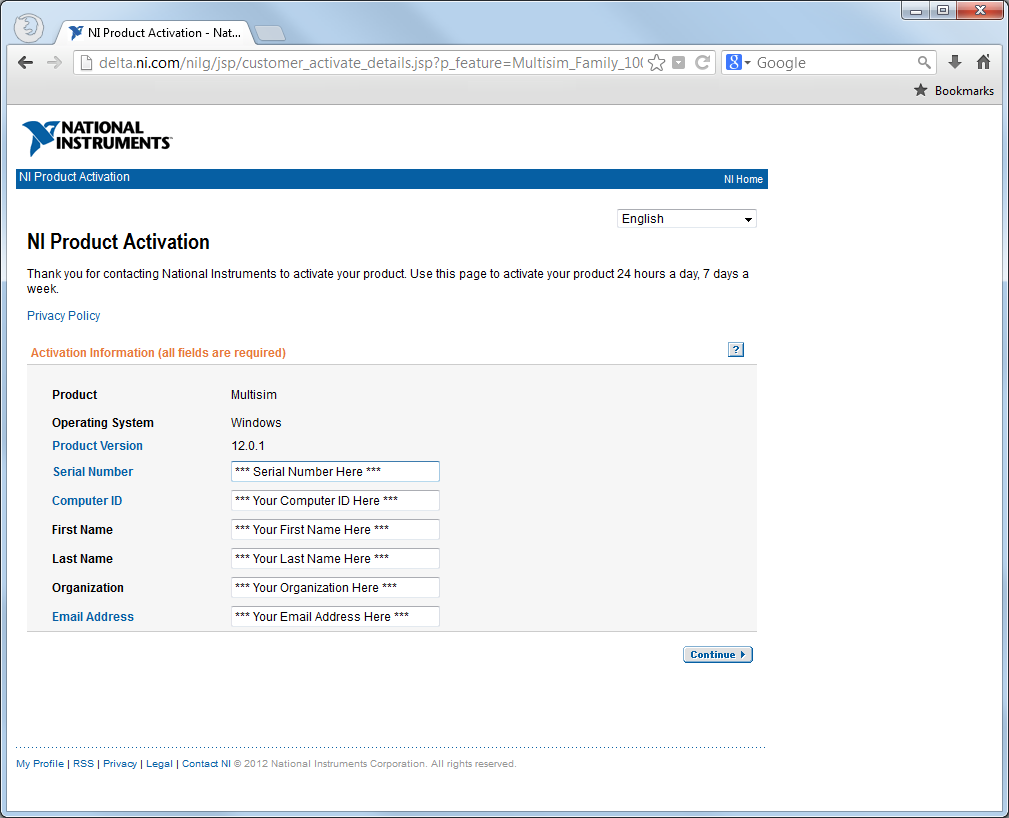The image shows a screenshot of a Firefox web browser running on a Windows operating system, reminiscent of Windows Vista due to its dated interface. The URL displayed in the address bar reads "https://delta.ni.com," and the browser tab is labeled "NI Product Activation."

The webpage itself belongs to National Instruments and features their blue logo prominently in the header. Under the header, the title "NI Product Activation" is displayed against a blue background that spans the width of the page, with the text in white. Below the title, a welcome message reads, "Thank you for contacting National Instruments to activate your product. Use this page to activate your product 24 hours a day, seven days a week," followed by a "Privacy Policy" link in blue text.

The main content of the page is an activation form. The section header "Activation Information" is highlighted in orange text. The form fields are listed with labels: "Product" with the value "Multi.ISM," "Operating System" with the value "Windows," "Product Version" with the value "12," followed by input fields for "Serial Number," "Computer ID," "First Name," "Last Name," "Organization," and "Email Address."

At the bottom right of the form, there is a "Continue" button for users to proceed with the activation process.